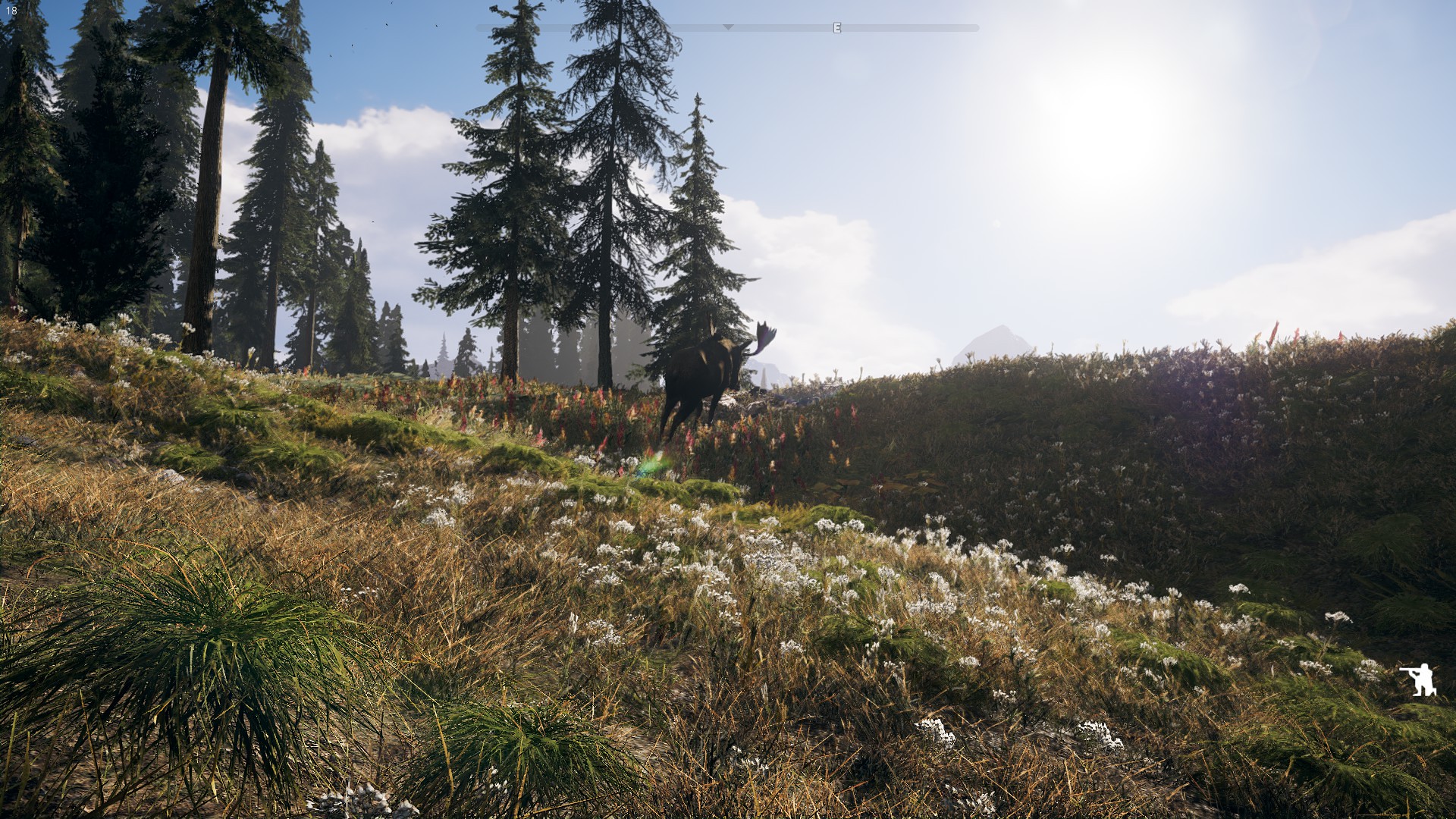This photograph captures a picturesque natural scene characterized by a field of overgrown grass interspersed with a variety of flora. In the foreground, a mix of white, green, and brown grass can be seen, peppered with tiny white flowers and scattered dandelions. Adding to the rich tapestry of the scene, yellow and pale red flowers bring splashes of color to the grassy landscape. 

In the background, verdant trees rise up, their green and brown hues contrasting beautifully against the blue sky. The sky itself is adorned with fluffy white clouds and the bright sun shining from one corner. A tiny white icon, reminiscent of a soldier crouching with a weapon, is subtly situated in one corner of the image, adding an intriguing, almost hidden element to the scene. This idyllic setting, filled with natural beauty and a hint of mystery, invites viewers to ponder and appreciate the simple wonders of the outdoors.